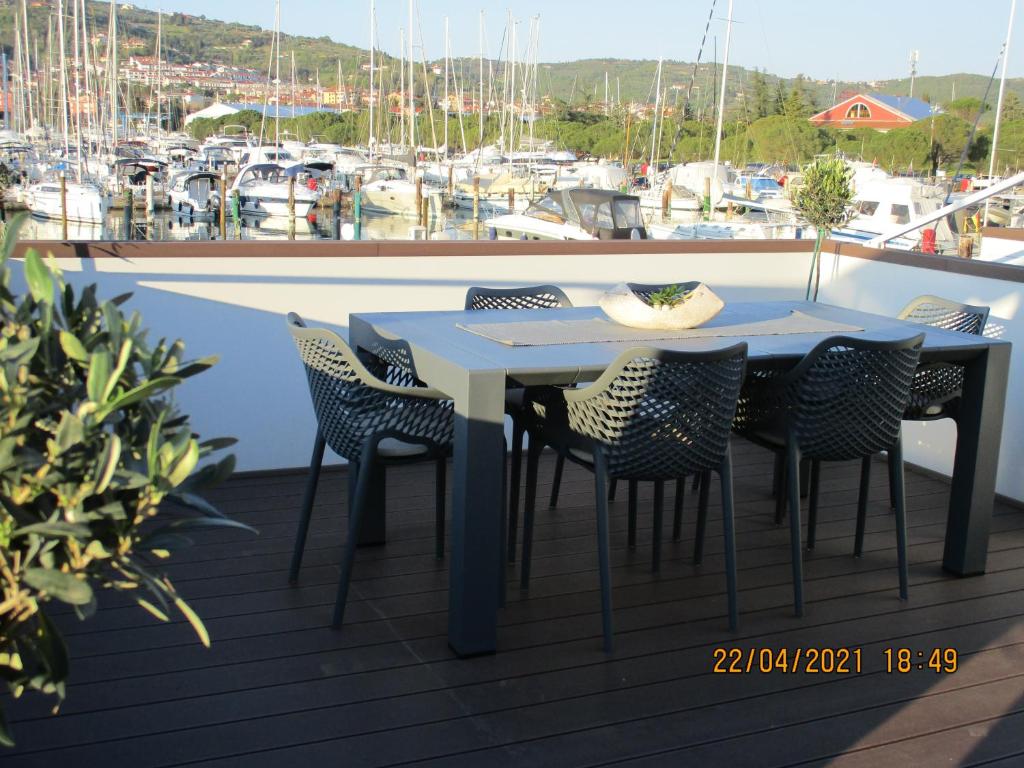The image captures a serene marina scene, featuring a dark wooden deck with a focal point of a square blue table with dark blue legs, surrounded by six matching blue wicker chairs. The deck is accessorized with a lush plant intruding from the lower left side of the frame. A short white wall with a brown edge encircles the deck area. The vibrant marina extends beyond the wall, densely packed with boats floating on the calm water. In the backdrop, a picturesque landscape unfolds with clusters of green trees and sprawling hills. Towards the upper left, there are hillside buildings and more water, while the upper right corner reveals the top of a house with a red and blue roof. The sky above is clear and blue, adding to the tranquil atmosphere. A timestamp in orange at the bottom right of the photograph reads "22/04/2021 18:49," documenting the moment this peaceful scene was captured.